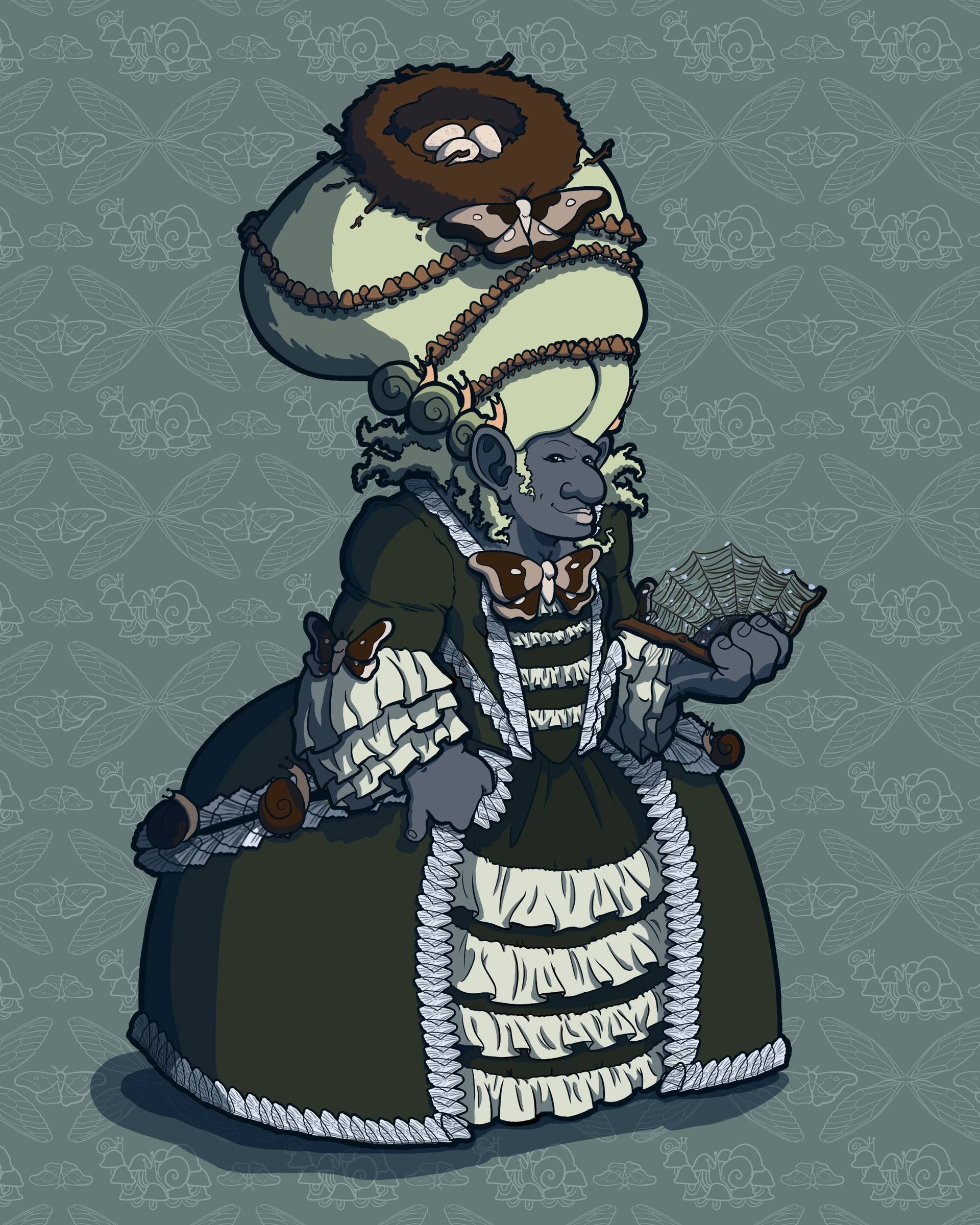The image depicts a detailed and elaborate cartoon drawing of a woman with an animalistic appearance, characterized by her gray skin tone and enormous ears. She wears an extravagant headdress that resembles a large white wig adorned with butterflies, beads, and even a bird's nest with eggs, emphasizing its size. Her facial complexion is gray, while other descriptions suggest a blue hue, adding to a possibly whimsical or gothic aesthetic. The woman is dressed in a lavish, old-fashioned colonial-style gown, reminiscent of the Martha Washington era, complete with ruffles, a petticoat, and a bow on the top. Her voluminous, floor-length dress, detailed with frilly fluffs at the bottom, hides her feet completely. She holds a fan in her left hand and clutches her dress with her right hand. The dress and accessories, including butterflies and decorative snails, contribute to the image's ornate, almost parodic or gothic vibe. The background is gray, enhancing the overall monochromatic and intricate design of this character.